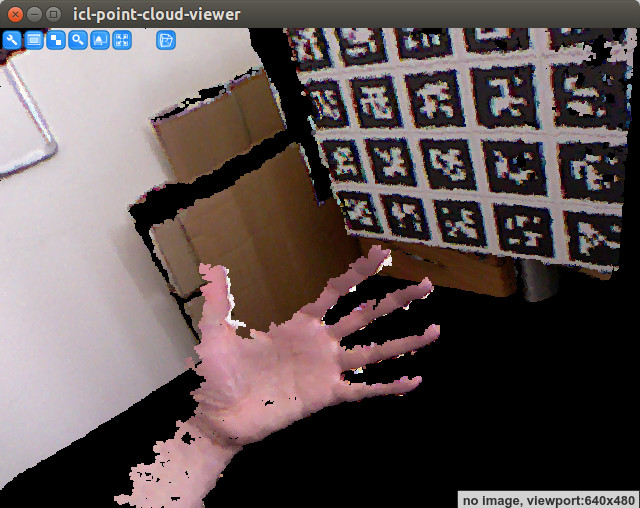The image features a detailed user interface of the ICL-Point-Cloud-Viewer. The top inch is dominated by a dark gray border. On the top right corner, there is a red circle with a gray 'X', a gray circle with a line across it, and another gray circle with a black square inside. These elements are likely buttons for closing, minimizing, and maximizing the window. The bold white text "ICL-Point-Cloud-Viewer" is prominently displayed below this border.

Underneath the header, there is a somewhat distorted image. Approximately two inches from the left edge, a wrist is visible, leading to an open palm with the thumb pointing to the left and the fingers pointing to the right. The hand is long, skinny, and slightly pixelated against the background. Surrounding the hand, the background is mainly black, with a cluster of black space about an inch to the left of the fingers and another cluster to the right.

In the top left corner, there are six blue squares arranged in a row, with a small space separating them from an additional blue square. Each square contains white icons, signifying different clickable options. Below this section, stretching from the left corner, is a white wall segment that extends upwards for about two inches before zigzagging towards the right. The wall's curving pattern and other elements depict some structural detail with cardboard material in the middle right section.

To the right of the central image area, the design appears to show five horizontal rows and four vertical columns of black squares adorned with what resembles Chinese writing. This design element adds an intricate background pattern to the wall.

In the bottom left corner of the interface, a gray tab displays "No Image, Viewport 640 x 480" in black text, indicating the image resolution or some additional view option.